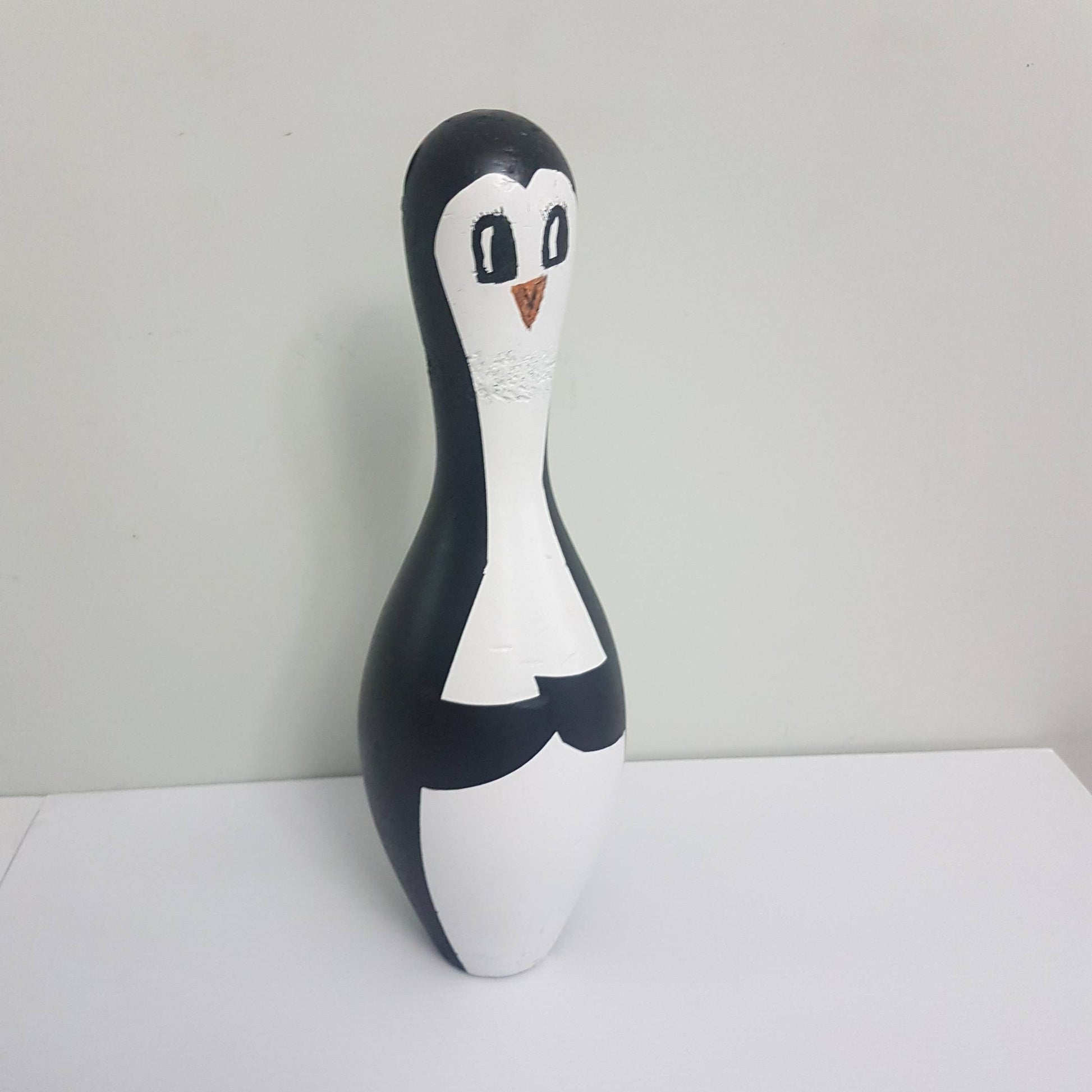The photograph captures a creatively painted bowling pin designed to resemble a penguin. The background features a light gray or white wall, and the pin is positioned on a flat white surface with a visible crease to the left, indicating that it is made up of two joined surfaces. 

The bowling pin itself has been intricately painted with a black and white design, showcasing an artistic transformation into a penguin. The top of the penguin, painted in black, forms a heart-shaped face with white details, tapering into a slimmer neck area that widens again towards the base. The eyes of the penguin are detailed with black edges and centers, giving it a lively expression as it gazes to the right. An orange, inverted triangle-shaped beak with hints of black further enhances its lifelike appearance. The penguin's front flippers, also black, are depicted as folded up in front of its body, adding a charming touch to the artwork.

The light source, coming from the right off-screen, casts a subtle shadow of the penguin slightly to its left. Notably, there are visible pit marks around the neck area of the bowling pin, adding texture and authenticity to the piece. Overall, the photograph beautifully captures the whimsical and detailed transformation of a simple bowling pin into a delightful penguin figure.